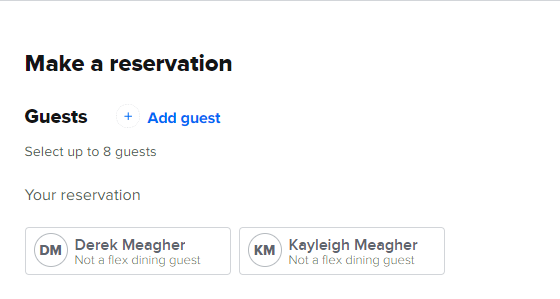The website interface for making a reservation prominently displays the heading "Make a Reservation" in large, bold black letters at the top left corner. Directly below this heading, the word "Guests" appears in bold black font, followed by a blue plus sign and the phrase "Add Guest" also in blue. In smaller print beneath, it informs users they can select up to eight guests. Below this section is the subheading "Your Reservation," accompanied by two white boxes outlined in gray.

The first box features a white circle with gray lining containing the initials "DM," along with the note "Not a Flex Dining Guest." The second box similarly displays a white circle with gray lining, containing the initials "KM" and the name "Kaylee Maker" underneath. This box also includes the note "Not a Flex Dining Guest." It appears that the reservation currently includes two guests, with an option to invite up to eight total guests, and the notation ensures the restaurant is aware that these individuals are not Flex Dining Guests in advance.